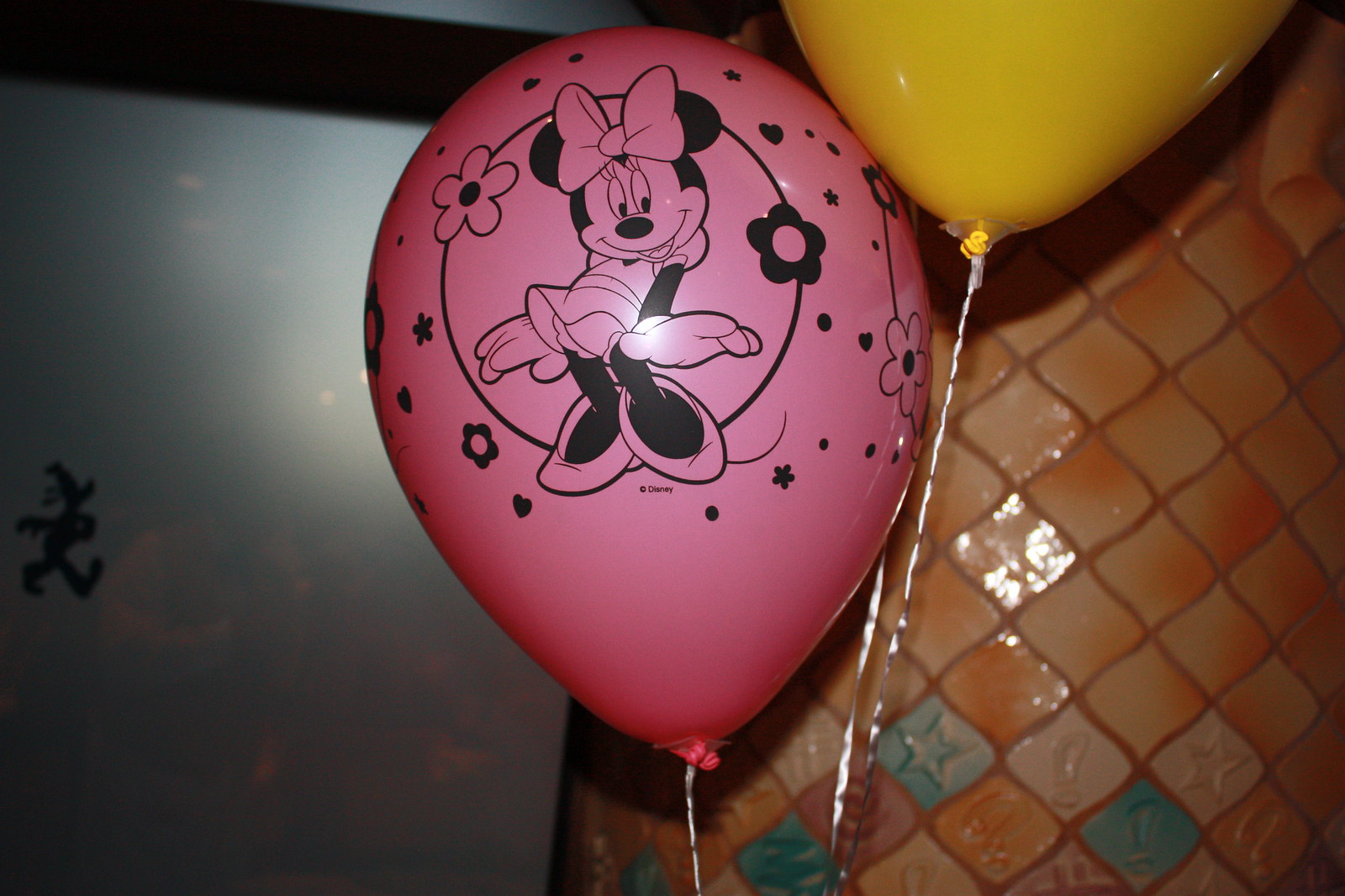The photograph is a detailed close-up image capturing a celebratory scene likely taking place indoors, possibly at a restaurant or a party. The central focus of the image is a pair of balloons: a pink balloon on the left, featuring a black and white portrait of Minnie Mouse encircled by a whimsical array of flowers and hearts, and a bright yellow balloon slightly higher and to the right. Behind these vibrant balloons, the background reveals a wall tiled with predominantly orange squares, interspersed with a few turquoise tiles adorned with stars and exclamation mark inlays, suggesting a visually engaging setting. To the left, there is an out-of-focus area that might be a doorway or mirror, highlighted by faint lights shining down from above and hinting at an ongoing celebration. The overall ambiance is warm with a mix of hues including black, white, light blue, pink, yellow, teal, maroon, and orange, enhancing the festive atmosphere.